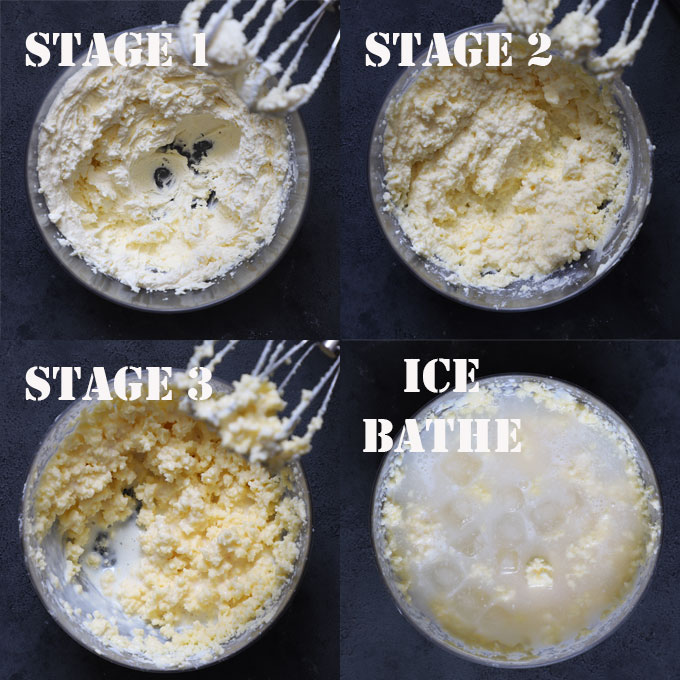This image presents a detailed four-stage process of making a dessert. In the top left corner, labeled "Stage 1," a bowl seen from above contains a white mixture being worked by two whisks positioned at the bowl's edge. Moving to the top right, "Stage 2" shows the same bowl with a thicker, more integrated mixture, still being stirred by the visible whisks. In "Stage 3," located in the bottom left, the mixture has transitioned to a chunkier, yellowish consistency with some of it caught in the whisks, which remain in the top right part of the frame. Finally, in the bottom right "Ice Bath" stage, the bowl now appears partially encased with a translucent covering, possibly indicating an ice bath step. The whisks are no longer present, and the mixture beneath the cover has a whiter, icing-like appearance.